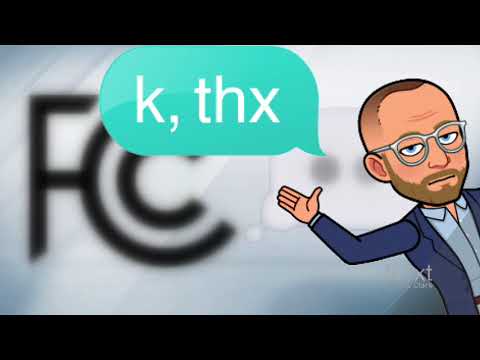The image is a computer-generated, color illustration with a landscape orientation, inset in a black background with black bars across the top and bottom. It depicts a man on the right side, appearing as if he is leaning or exiting the frame, with his hand raised in a gesture that could be interpreted as waving or pointing. The man has very short, partially translucent gray hair, a peach-colored complexion, and wears white-framed, gray-colored glasses. His eyes are partially open, showing just the top of his blue irises. He sports a full brown beard and mustache and is dressed in a dark blue blazer over a light blue shirt. 

His slightly open mouth is represented as a black line, and he appears to be speaking into a teal-colored speech bubble that contains the text "k, thx" in lowercase letters. The background behind him is predominantly white with a blurry black FCC logo, characterized by a large 'C' with a smaller 'c' underneath it. The image conveys a modern, illustrative style with a conversational and somewhat casual tone.